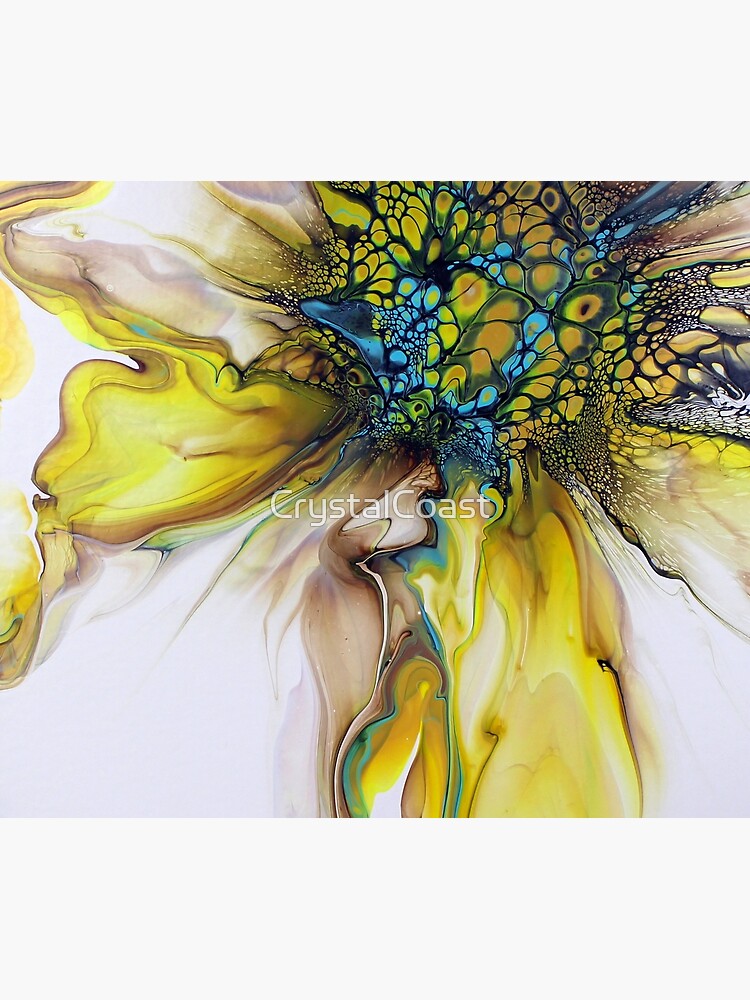The image showcases a striking digital artwork resembling a large, abstract flower, painted with watercolor or oil paints in a minimalistic style. The flower's petals, which are predominantly yellow with hints of white, gold, brown, and blue, appear to radiate outwards from a dark blue center accented with darker yellow and black splotches. The center itself includes intricate details of seeds and circular patterns. The background is solid white, bordered by a light gray, almost off-white thick frame at the top and bottom. Across the center of the image, the text "Crystal Coast" is prominently displayed in white letters. The overall effect is reminiscent of a splatter painting, with colors spreading dynamically towards the edges, creating a vibrant and eye-catching composition.